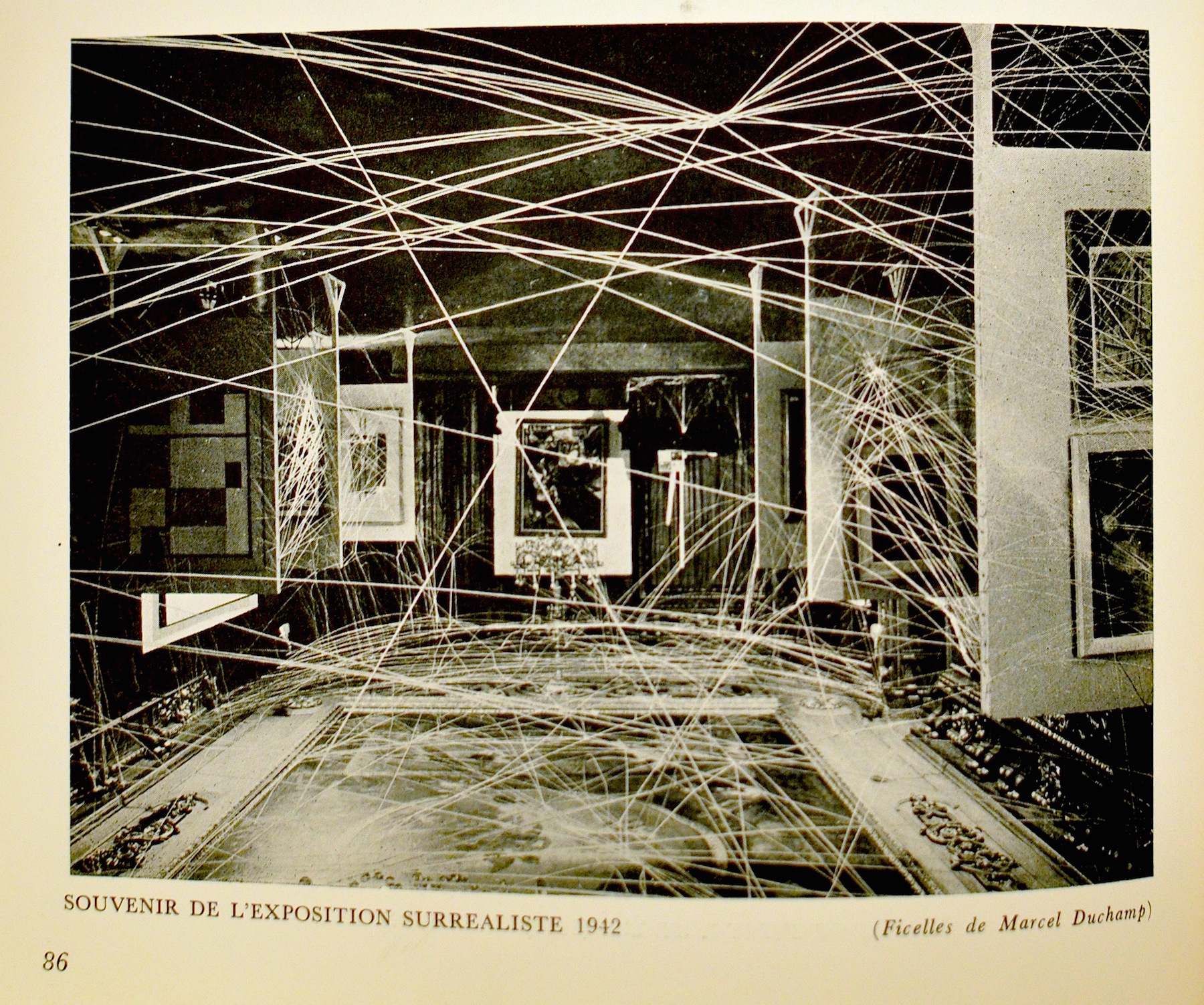The photograph showcases a sepia-toned postcard from 1942 labeled "Souvenir de l'Exposition Surrealiste 1942," attributed to the artist Marcel Duchamp. The image depicts an art gallery adorned with various paintings and photographs. Suspended throughout the space are strings or lines that crisscross from floor to ceiling and wall to wall, reminiscent of laser security in a heist movie scene. The intricate web of lines might either be physical strings or an artistic overlay added after the fact. The foreground of the image features some scratches, suggesting the photograph's age and wear. The photograph is printed on an off-white, yellowing page, with "Faciles de Marcel Duchamp" inscribed, along with the page number 86 in the bottom left corner.